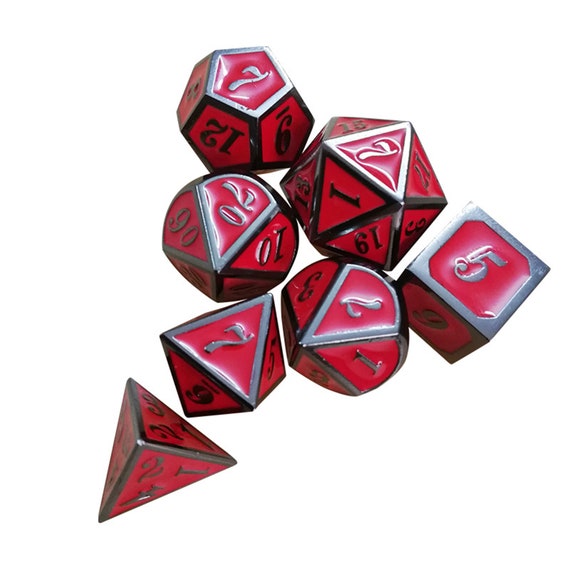The photograph showcases a collection of seven gaming dice arranged in a roughly triangular formation. The dice are predominantly red with metallic accents, featuring numbers in silver, black, or pewter-colored fonts. The collection includes a variety of shapes: a traditional six-sided die, several triangular or pyramid-shaped dice, and others with more complex geometries, such as a 12-sided die. These dice are all crafted with a glossy, metallic finish, adding an elegant sheen to their surfaces. Some of the dice display unique numbers like 12, indicating a higher number of sides. The combination of different shapes and color schemes provides a visually striking and detailed array of gaming dice.